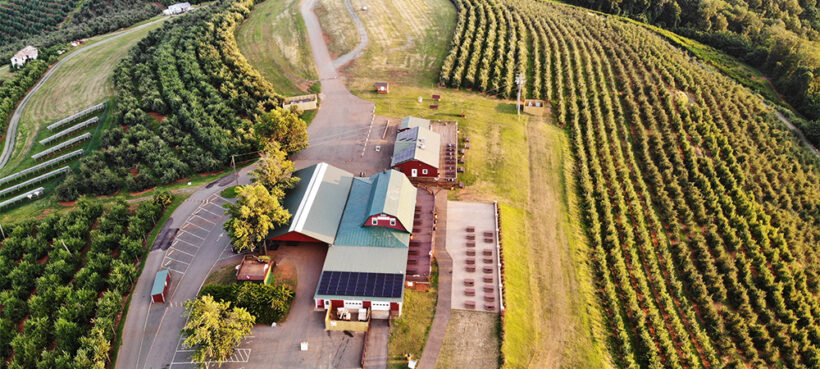A high-resolution satellite image of a sprawling hillside farm captures a detailed aerial perspective. The farm, situated prominently on the hilltop, comprises three large buildings with white roofs that stand out vividly, suggesting possible photo-enhancement. Surrounding these structures are additional outbuildings and ample parking spaces, indicating a substantial operational scale. The farm is flanked by expansive asphalt roads, including a notable fork branching off to different directions. The land directly adjacent to the farm reveals meticulously arranged rows of cultivated crops, potentially grapes or similar produce, extending across much of the visible terrain. To the left of the main cultivated area, an orderly series of tree rows further enriches the agricultural landscape. The entire scene epitomizes a well-organized and thriving farming enterprise.